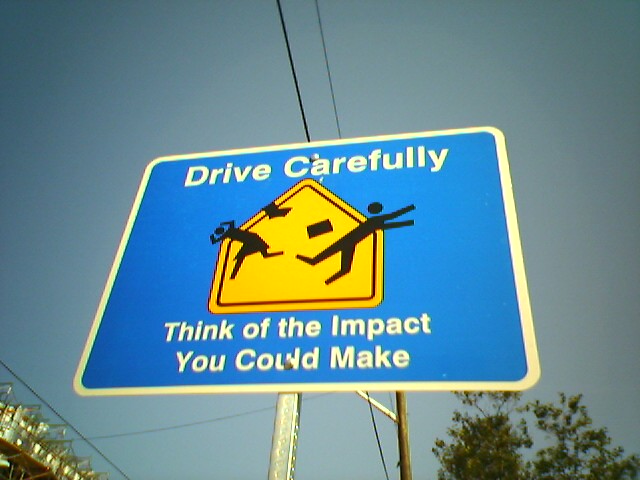This image showcases a road sign, photographed from a low angle, emphasizing the upward perspective from the base to the top of the sign. The sign is mounted on a visible portion of a pole. Dominating the image, the blue sign features a prominent white border and consists of several distinct elements.

At the top, the sign displays a cautionary message in white font: "Drive Carefully." Below this text, in the center, there is a yellow silhouette of a house. Flanking the house, illustrations of people appear to be jumping away, each seemingly tossing a book into the air.

Finally, towards the bottom of the sign, another phrase in white text reads: "Think of the impact you could make." The combination of the imagery and text serves as a striking visual reminder for drivers to be cautious on the road.